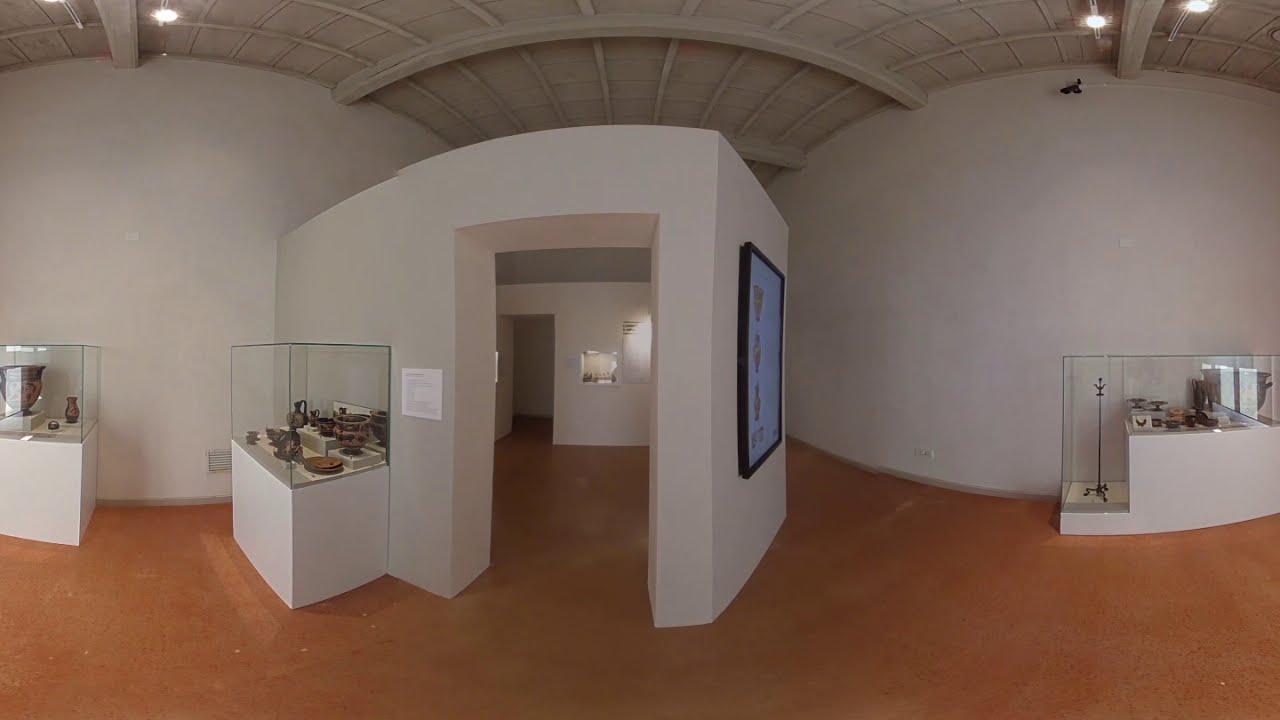The image depicts a modernist museum interior with curved, off-white walls and ceiling, complemented by an orangish-brown wooden floor. Throughout the foreground and background, there are white-base display cases with glass tops, housing various valuable objects. To the left of the room, next to the main doorway, lies a series of white and glass showcases containing brown-colored items, possibly pots or artifacts. The same type of showcases are visibly placed along the right wall, each holding different items. The ceiling, featuring visible wooden rafters and arch support structures, has a beige hue and is adorned with multiple hanging lights positioned at the top left and right corners. The center of the photo highlights a white, doorless entryway leading to another similar doorway. There are small plaques and signs adjacent to the displayed objects, suggesting informative descriptions or titles, enhancing the museum atmosphere.